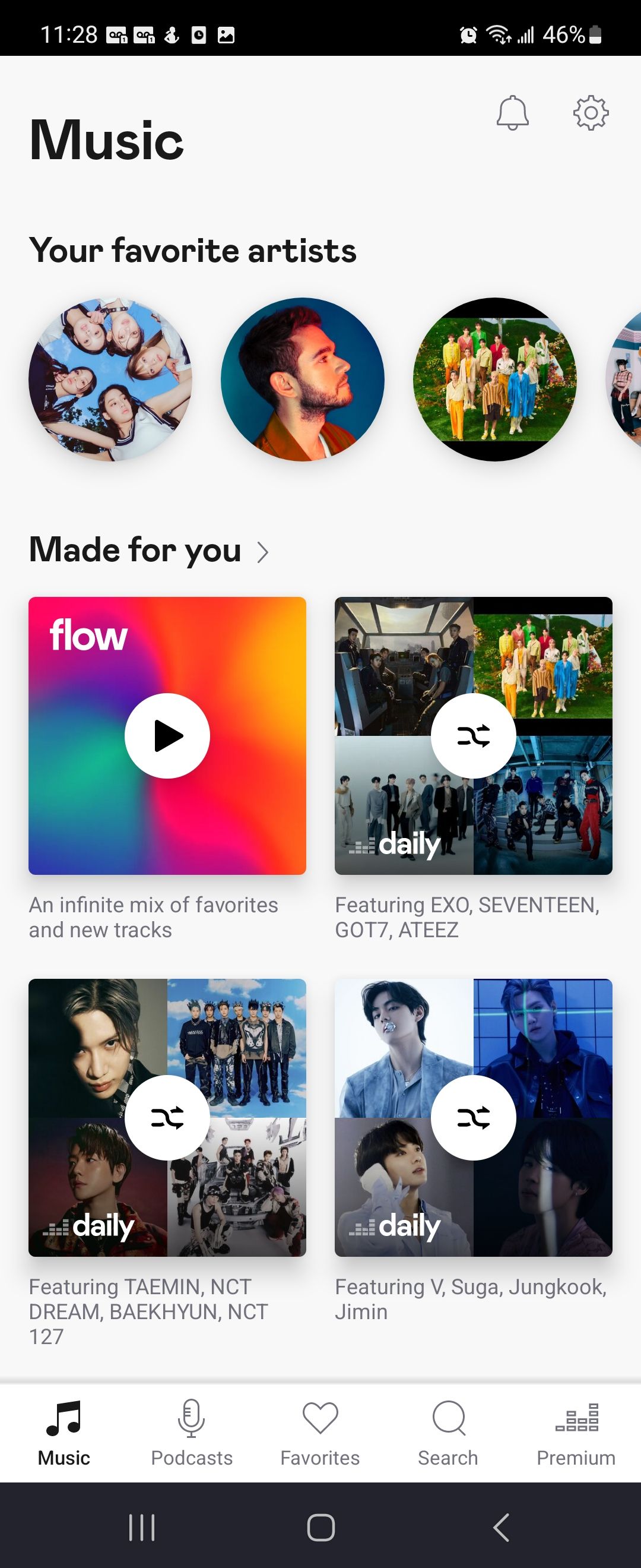A detailed screenshot of a mobile phone display is shown. At the top of the screen, a black status bar features white font showing the time as 11:28. To the right of the time, there are five square icons with small symbols inside, followed by icons for an alarm clock, Wi-Fi signal, and mobile data. The battery percentage is displayed as 46% next to a battery icon.

Directly below the status bar, the screen has a white background with “Music” written in bold black font. To the right of the word "Music," there are a small gray bell icon, likely for notifications, and a gray gear icon for settings. Beneath this, it says "Your Favorite Artists" in black font.

The section below features three circular images depicting the user’s favorite artists. The image on the left shows five Korean women looking downwards. The middle image is of a Black man facing right, wearing a red shirt. The image on the right shows a group of people standing on a hill.

Further down, "Made for You" is written in black font, followed by various playlist options. One of the playlists is labeled "Flow."